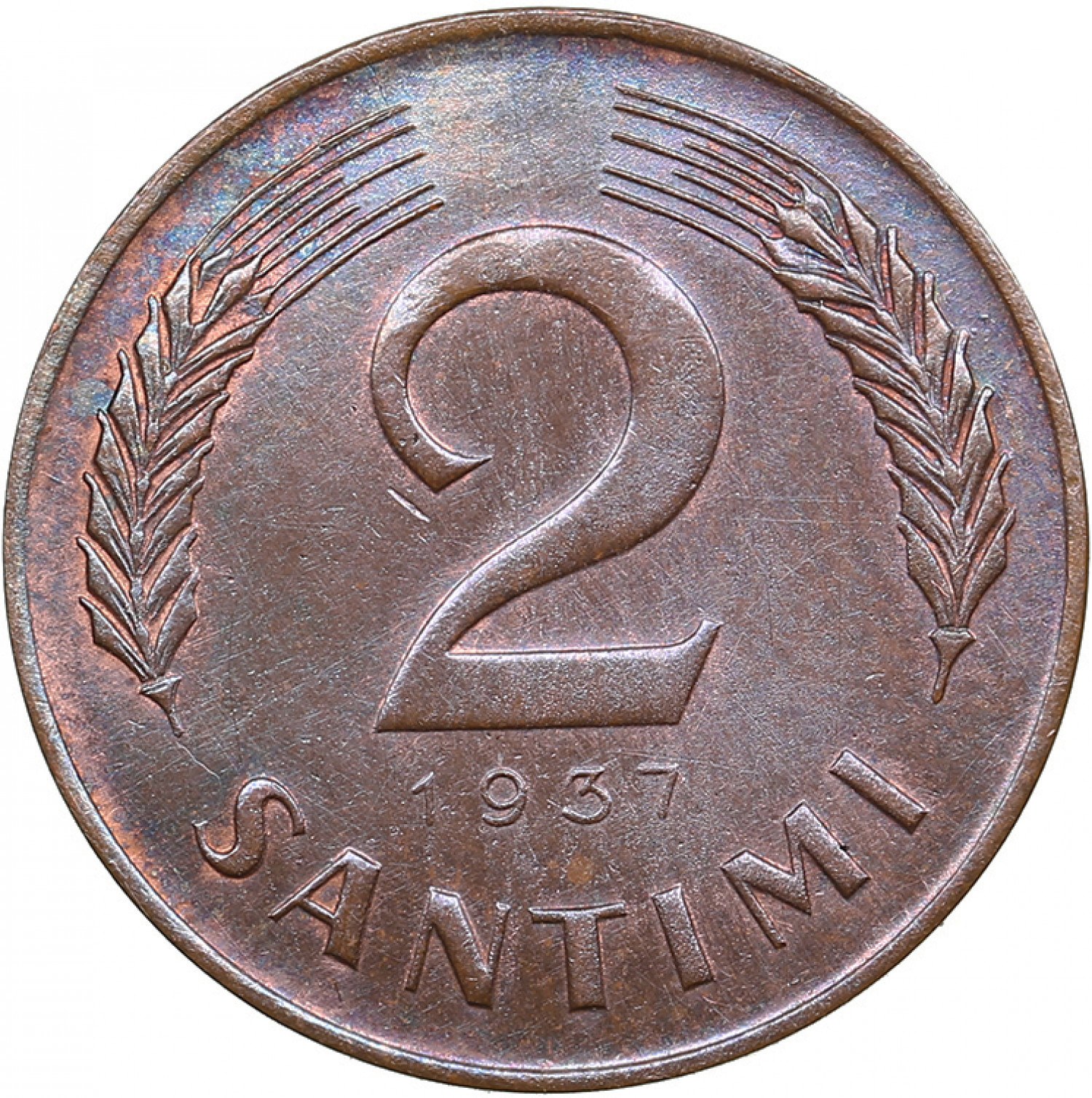This detailed image captures the reverse side of a 1937 coin, set against a white background. The coin, which appears to be composed of copper or bronze, exhibits a reddish-brown surface with a shining luster that intensifies in its crevices, particularly highlighting areas like the center of the "A" and the grooves of the wheat stalks. Dominating the center of the coin is a large numeral "2," flanked on either side by curved strands of wheat, which together create a near circular frame. Beneath the numeral "2," the date "1937" is prominently displayed, followed by the word "SANTIMI" in block capitals, curving gracefully with the wheat strands. The coin features a slightly raised rim and includes a small etched line on the left side of the numeral "2," indicating its aged and well-worn condition.